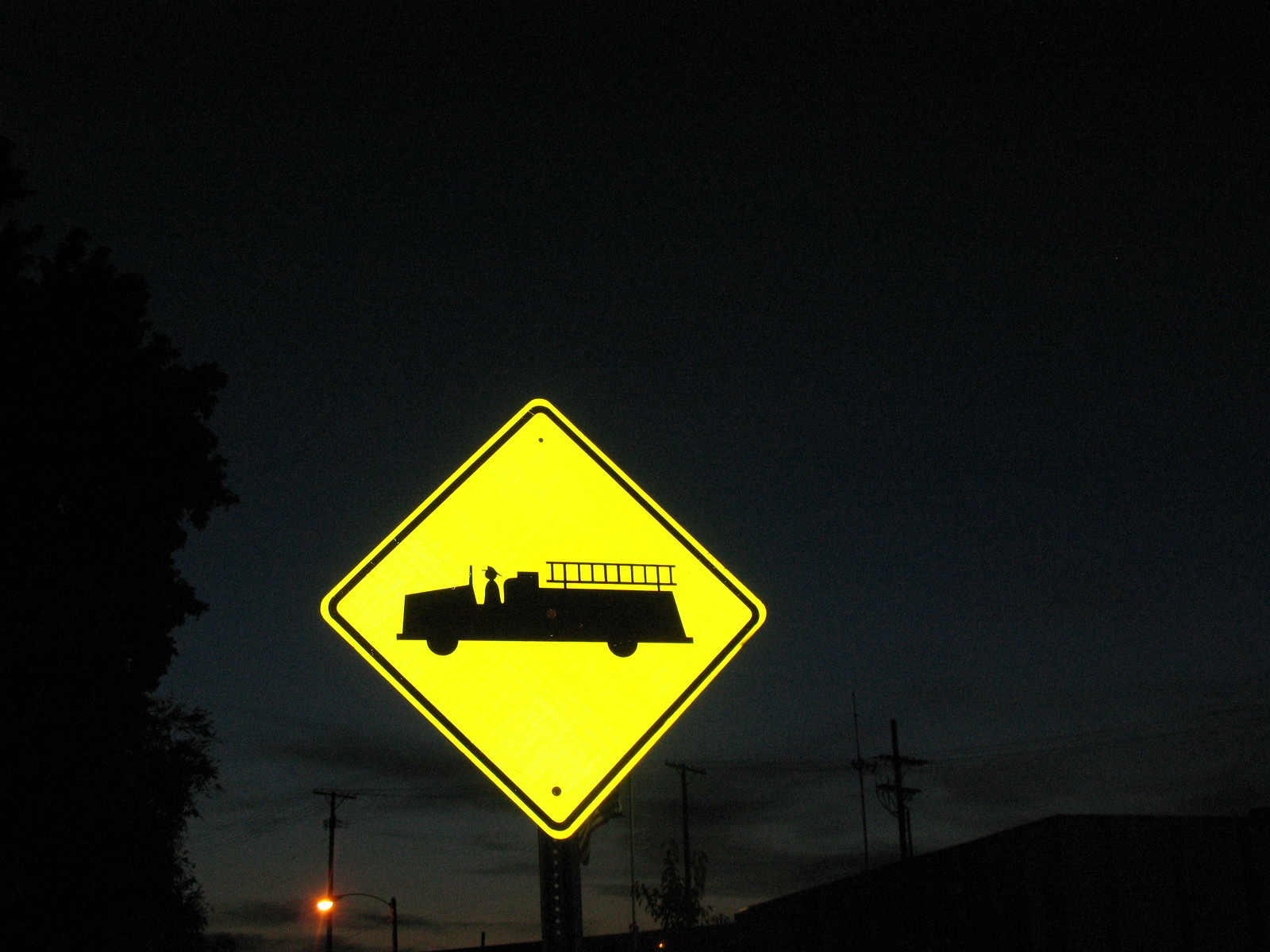A nighttime photograph captures a diamond-shaped, yellow signpost with a black border near its edge. At the center of the sign, an illustration depicts a firefighter riding in a fire truck. The dark sky in the background indicates that the picture was taken after sundown. The sign is brightly illuminated, likely due to the camera's flash, which reflects off the sign's surface.